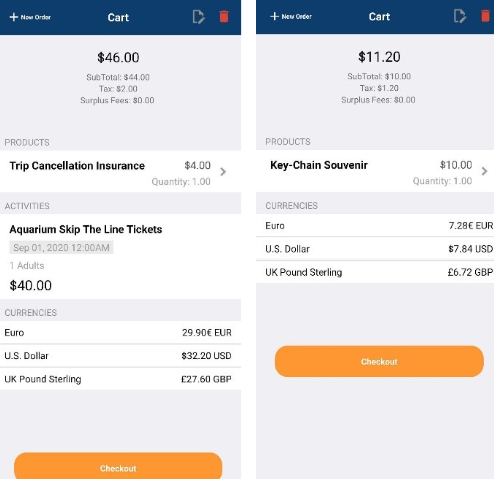The image depicts two digital screens, side by side, displaying transaction details for different purchases.

### Left Screen:
1. **Top Section:**
   - A blue rectangle with an unclear symbol and some indecipherable text, along with a cart icon.

2. **Details Section:**
   - **First Item:**
     - A gray rectangle displaying the amount: "$46.00".
     - Unclear text beneath this amount.
   - **Second Item:**
     - A white rectangle labeled "Trip Cancellation Insurance: $4.00".
     - An arrow pointing to the right, with more unclear text below it.
   - **Third Item:**
     - A gray rectangle labeled "Activities".
     - A white rectangle labeled "Aquarium, Skip the Line Tickets".
     - A gray rectangle underneath, showing the date information (indecipherable), and stating "One Adult: $40.00".

3. **Currency Section:**
   - A gray rectangle labeled "Currencies".
   - Listings for:
     - Euro (price in euros)
     - U.S. Dollars (price in dollars)
     - U.K. Pound Sterling (price in pounds)
     
4. **Checkout:**
   - A gray rectangle at the bottom with an orange button labeled "Check Out".

### Right Screen:
1. **Top Section:**
   - Similar to the left screen, featuring a blue rectangle with a cart icon and unclear text.

2. **Details Section:**
   - **First Item:**
     - A gray rectangle displaying the amount: "$11.20".
     - Unclear text beneath this amount.
   - **Second Item:**
     - A white rectangle labeled "Keychain Souvenir: $10.00".
     - An arrow pointing to the right, with more unclear text below it.

3. **Currency Section:**
   - A gray rectangle labeled "Currencies".
   - Listings for:
     - Euro (amount in euros)
     - U.S. Dollars (amount in dollars)
     - U.K. Pound Sterling (amount in pounds)

4. **Checkout:**
   - A gray square at the bottom with a prominent orange button labeled "Check Out".

Each screen offers detailed breakdowns of items for purchase, inclusive of prices in various currencies, and corresponding checkout options.